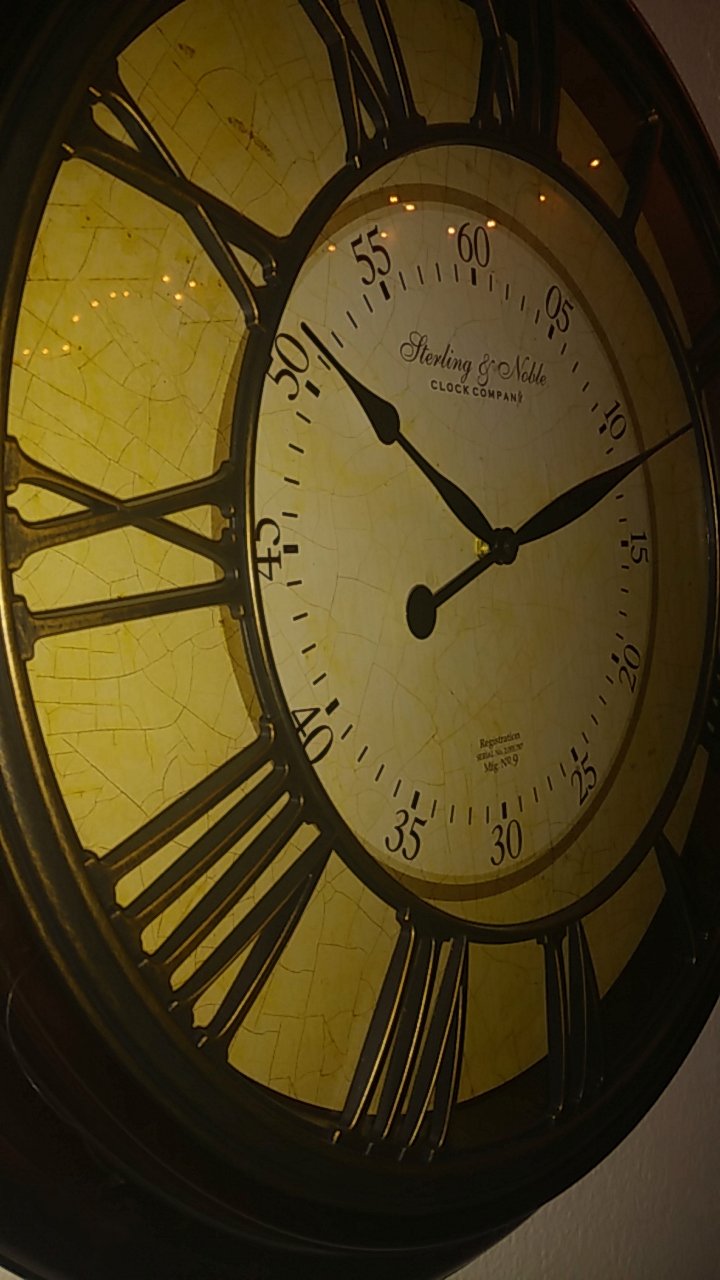This side-view photograph features a large, intricately designed clock. The outer edge displays Roman numerals marking the hours, crafted from a bronze-like metal that lends a classic and elegant appearance. Surrounding the clock face are standard minute indicators at five-minute intervals, labeled 60, 05, 10, 15, 20, 25, 30, 35, 40, 45, 50, and 55, with finer tick marks in between, providing precise timekeeping detail. At the center of the clock are regular Arabic numerals. The hands of the clock, robust and well-defined, point to approximately 10 and 2, indicating the time with clarity. The juxtaposition of Roman and Arabic numerals adds a unique, multi-layered visual appeal to this striking timepiece.